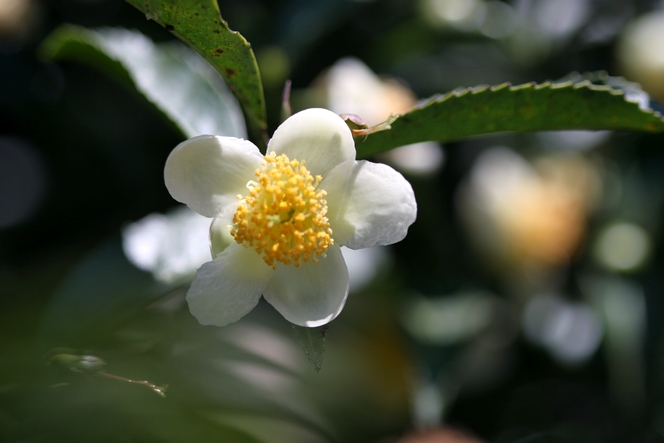This horizontally-oriented photograph captures a prominently featured white flower with a vibrant yellow center, surrounded by six delicate petals. The flower is shot with a bokeh effect, making its surrounding background of green, white, and yellow splotches indistinct and blurred. Above the flower, there's a serrated green leaf with some visible spots, likely from bug damage. More greenery and possibly additional flowers can be seen faintly behind the main subject. In the lower left-hand corner of the image, there is a small stem or leaf that adds to the natural setting. The overall focus of the image highlights the striking beauty of the white flower amidst a soft, dreamy background.